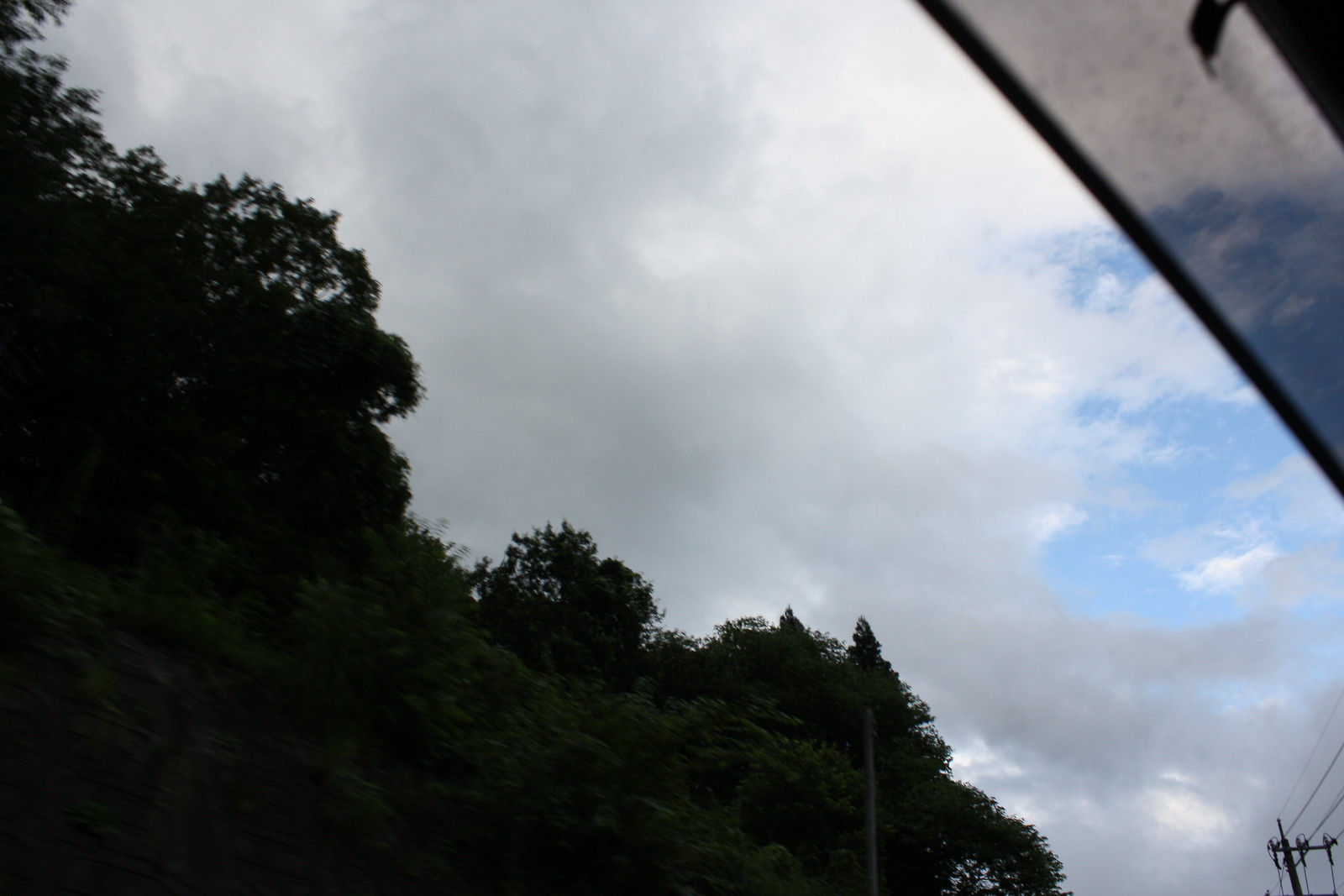The image captures an outdoor scene predominantly showcasing a cloudy sky filled with varying shades of gray and white clouds. The sky, which spans across the entire photo, has a slightly blue tinge amidst the gray. Taken from an angled perspective, approximately 45 degrees clockwise, there's an indication that the photo might have been shot from inside a car, suggested by the darkened, possibly tinted, sun shield visible at the top right corner. In the bottom right of the image, there are power lines and a pole with cables extending across the scene, affirming the outdoor setting. The left side is populated with a dense collection of dark green trees, creating a stark contrast against the cloudy sky. These tall trees are partially cut off by the photo’s frame. Additionally, there’s a hint of a rocky or cliff area in the lower left corner. The lighting suggests that the photo was taken during the daytime, but the extensive cloud cover imparts a darker ambiance to the scene. Overall, the image provides a comprehensive view of nature intersecting with human elements, framed by the perspective from a car window.